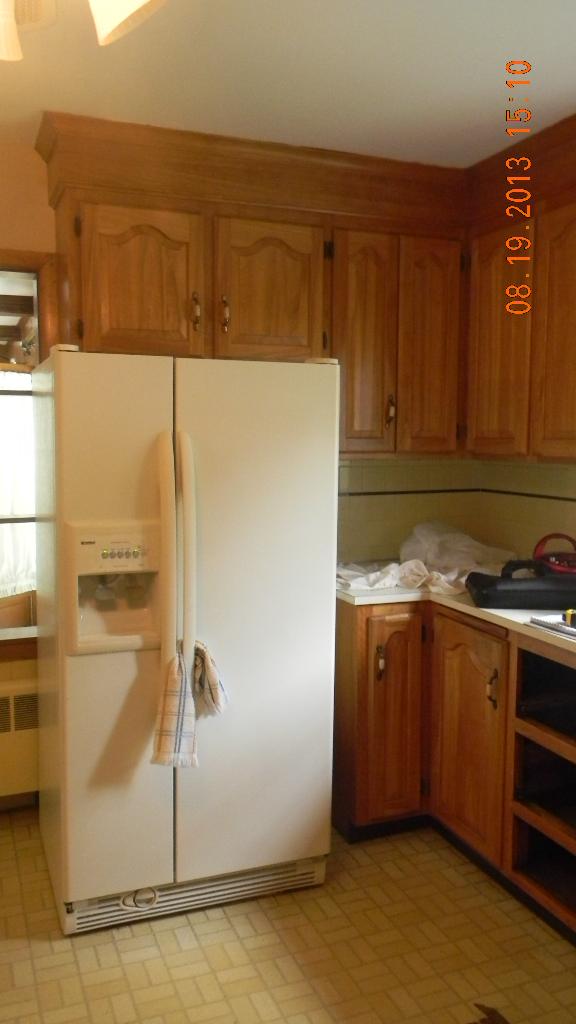The photo depicts a kitchen with a distinctly 90s aesthetic, captured on 08-19-2013 at 1510 hours. The room features both upper and lower wooden cabinets, possibly made of light brown or red oak. The floor is covered in a creamish yellow linoleum with capsule-shaped designs. There's a large, white side-by-side refrigerator freezer combination with a water and ice dispenser equipped with silver buttons facing the camera. A towel is tied around the refrigerator handles, and it appears slightly pulled away from the wall, though it may be an illusion. The white countertops are cluttered with various tools, fabrics, and containers, indicating either ongoing renovation or general messiness. In the background to the left, there's a window with a white curtain, and below it lies a vent, possibly a heater or air conditioner system. The kitchen is illuminated by daylight streaming through the window.